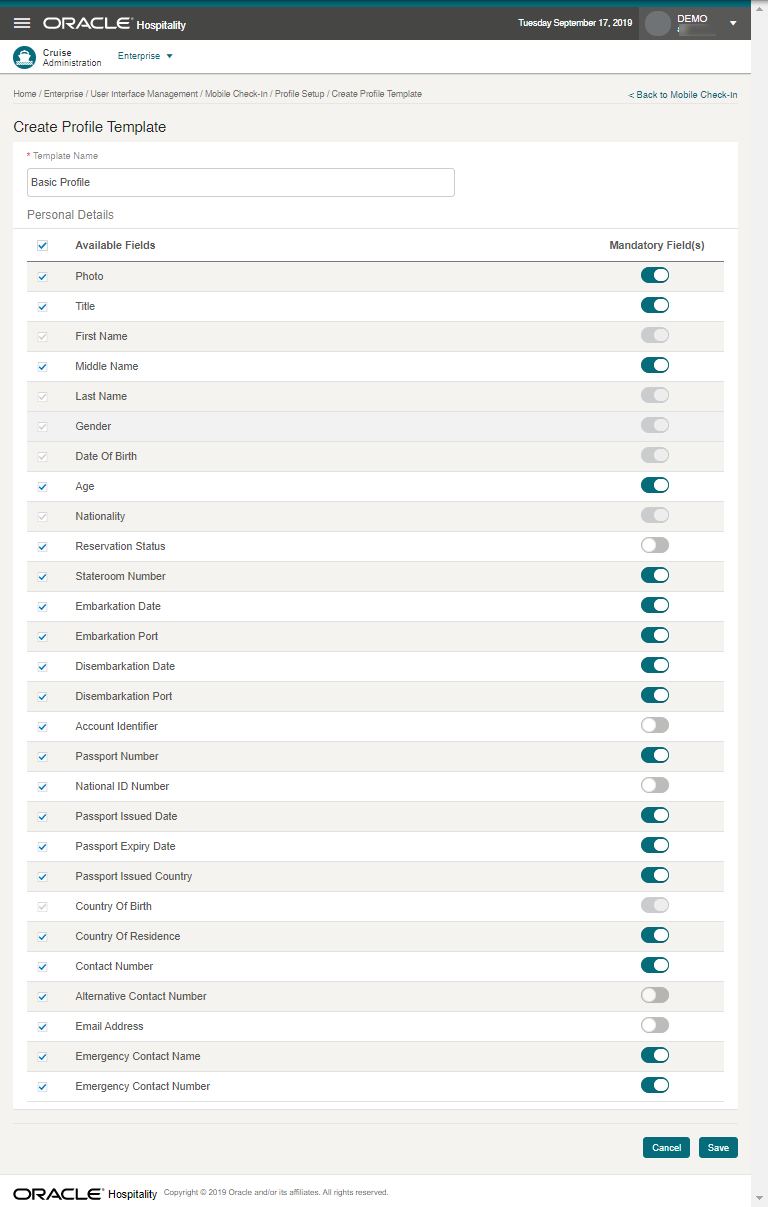A detailed screenshot depicting an Oracle Hospitality interface, potentially within an admin panel or back-end application. The top text of the screen reads "Oracle Hospitality," and on the upper right corner, the date is clearly marked as Tuesday, September 17, 2019. The system is currently logged in under a demo account. The main content area features an extensive list titled "Create Profile Template." Among the items listed, "Basic Profile" is highlighted as the template name, accompanied by various fields related to personal details that need to be filled in. Notable fields include mandatory entries such as "Photo," "Title," "Full Name," and other essential information like "Gender," "Date of Birth," "Country of Birth," and "Contact Number." Some fields have toggles allowing user-defined settings, while others are permanently set to mandatory, providing a comprehensive system for managing user profiles.